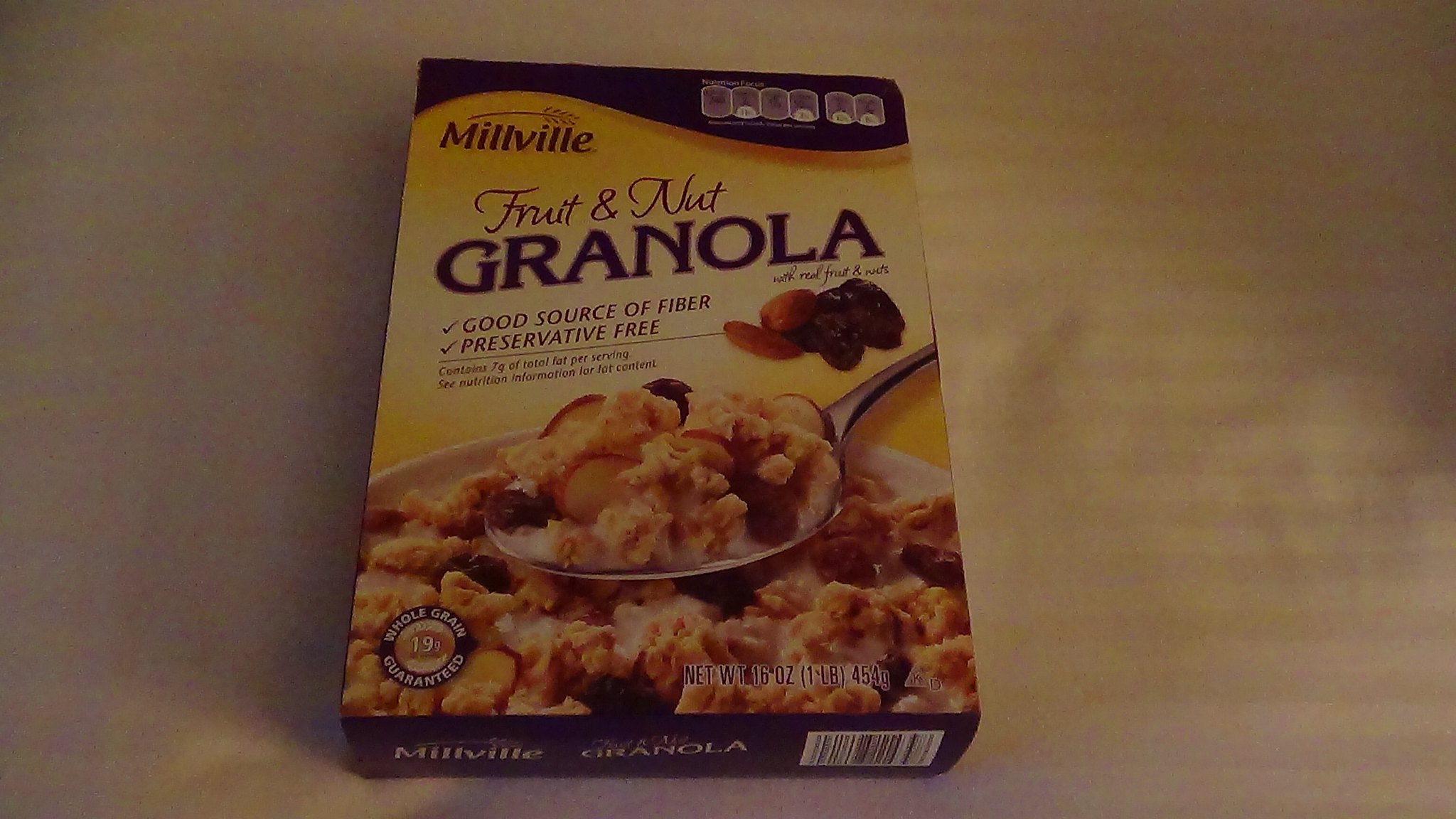The image showcases a box of Millville Fruit and Nut Granola. The box features a yellow background with a blue swirl at the top and a purple section for nutritional quick facts. At the top left, the Millville brand logo is displayed along with a wheat stem. Below the logo, the label reads "Fruit and Nut Granola" with an annotation of "with real fruit and nuts." Further down, checkmarks highlight statements like "Good Source of Fiber" and "Preservative Free." The box also notes, "Contains 7 grams of total fat per serving. See nutrition information for fat content." The net weight is specified as 16 ounces (1 pound). The design includes an image of a white bowl filled with the granola, featuring tan and brown cereal pieces, black raisins, and possibly almonds. A silver spoon is shown scooping the granola. This bowl is placed on a table or countertop with a tan cloth bearing brown stripes. Additional product information and a black-and-white barcode are visible at the bottom of the box.